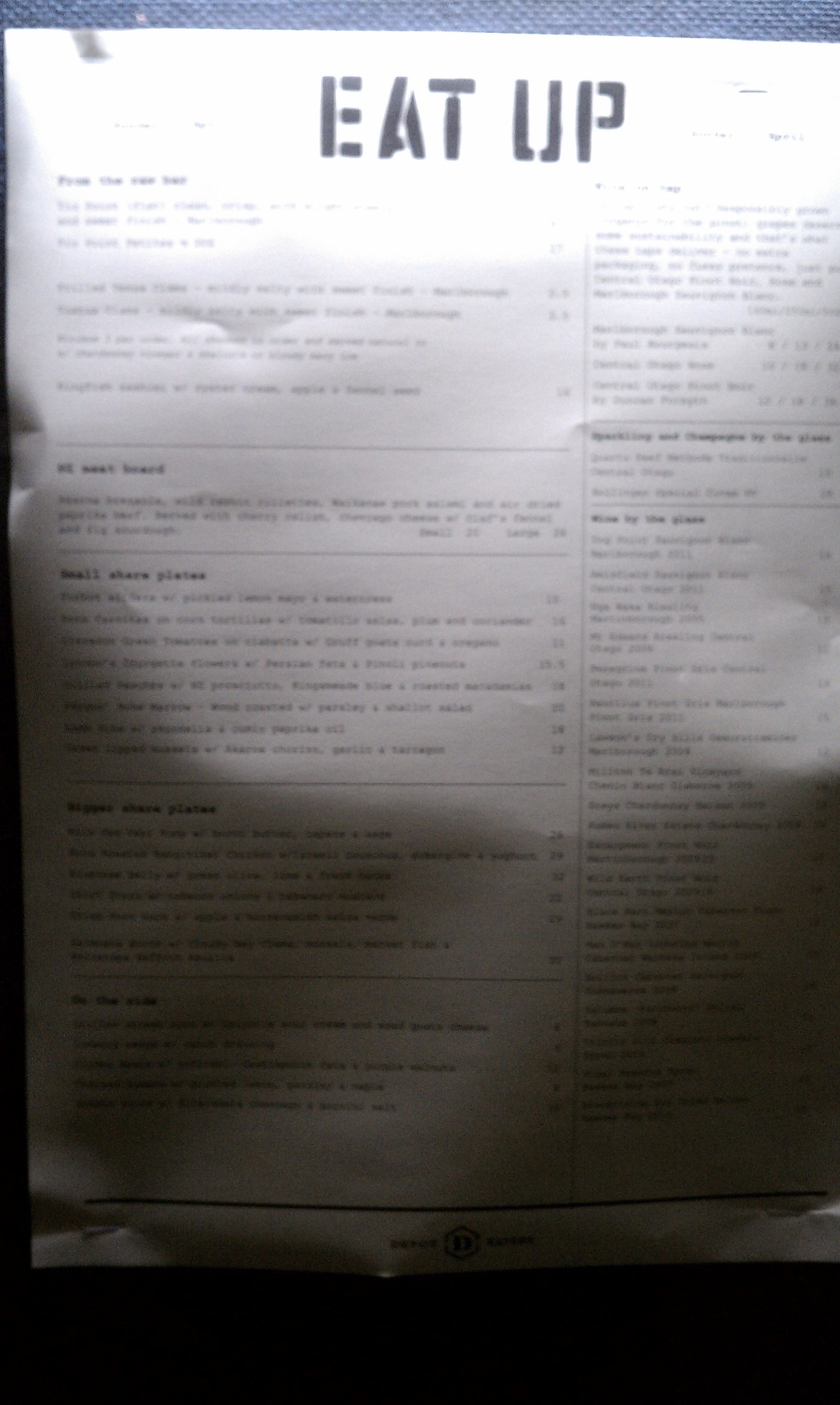A dimly lit restaurant menu captures attention with its unique, though imperfect, presentation. At the top, the header "Eat Up" is prominently displayed in bold black letters. The upper portion of the menu is bright white, providing a stark contrast to the bottom half, which is shrouded in shadow due to a shading error. The overall lack of focus further muddles the scene. The layout of the menu resembles a rectangular grid with various sections, including titles lined up on the left. However, the text throughout the menu is difficult to read, partly because of an overly glossy finish that makes it appear too shiny.